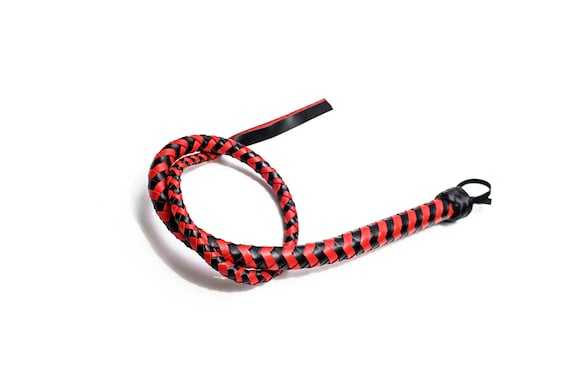The image showcases a black and red striped cord, neatly placed against a completely white background. The cord appears somewhat short and is tied into a loose, open knot, forming a loop at one end which could be used for holding or hanging. The material of the cord is shiny, possibly plastic, and it has a woven texture. One end features long, straight pieces of red and black strands, almost resembling a tassel, hanging freely. The cord starts from the middle right of the image, curls upon itself twice, and extends towards the top middle, creating a visually striking arrangement with its horizontal black and red stripes forming arrow-like patterns.